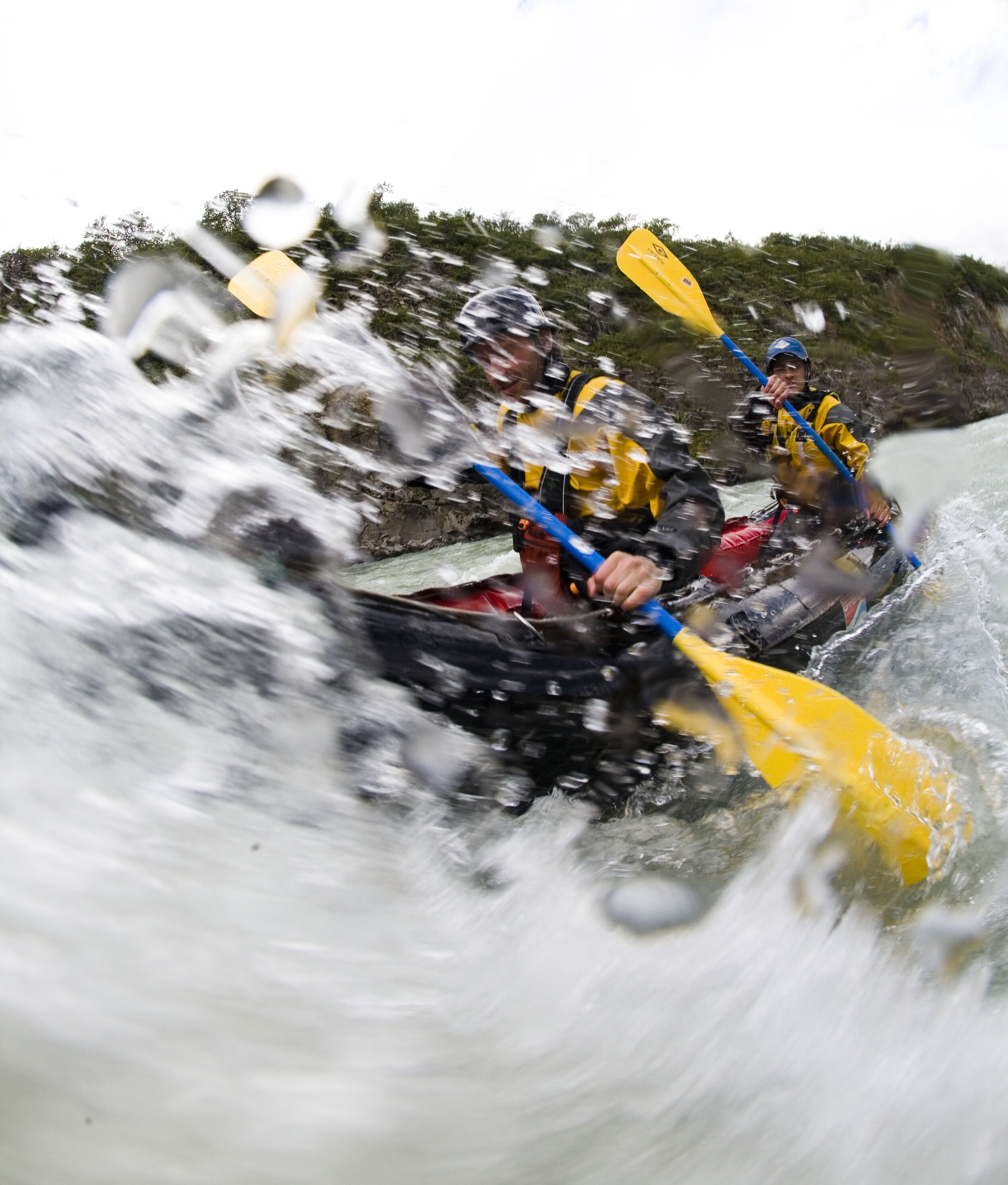This is a vertically rectangular, full-color photograph capturing an action-packed moment of two whitewater rafters in a kayak on a not-so-sunny day. The scene is set outdoors with a gray, overcast sky forming the topmost part of the image. Below the sky, a brownish-green embankment with sparse trees is visible. Dominating the left and bottom sections of the image, turbulent water splashes vigorously, obscuring the faces of the rafters.

The kayak, appearing to be black with a red interior, is in the center of the frame, pointed toward the lower left corner. Both rafters are wearing yellow life jackets with black trim, and they each hold double-sided paddles featuring blue handles and yellow blades. The man in the back sports a blue ball cap, while the details of the man in the front are mostly hidden by the splashing water.

The dynamic splash of whitewater, with droplets visibly suspended in mid-air, creates a dramatic foreground. Meanwhile, the calmer light-gray waters and the greenish embankment in the background provide a contrasting backdrop, amplifying the intensity of the moment captured in this photograph.